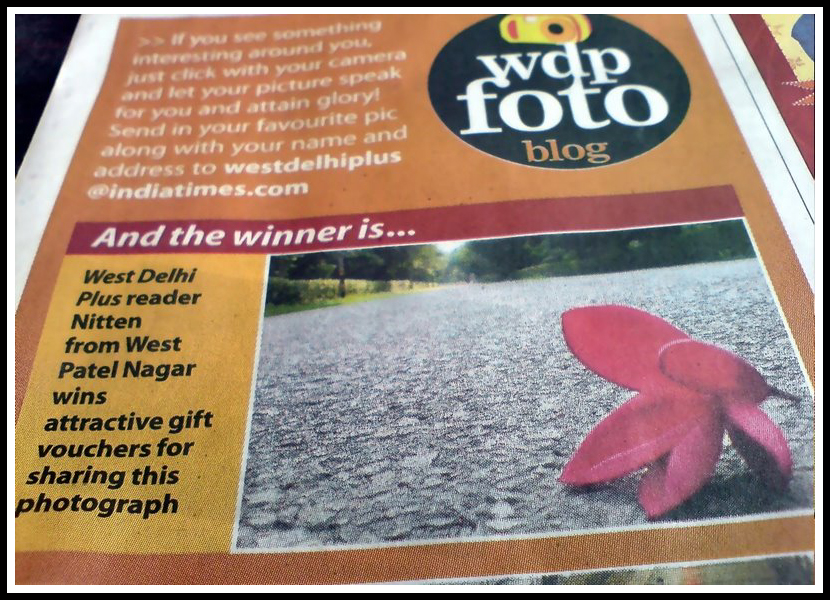The image showcases a detailed color print advertisement from a magazine, specifically from the left side of an open spread. Dominated by vibrant orange and gold hues, the page features a white-bordered layout. The top section of the page includes a nine-line paragraph of white text aligned to the left. Adjacent to this is a black circle featuring a yellow camera icon and the text "WDP Photo Blog," with "Foto" spelled out phonetically (F-O-T-O).

Below this, a prominent red strip with white text announces "And the winner is..." The photograph that follows covers the right two-thirds of the next section, depicting a gray road surface with a five-pointed star-shaped pink blossom or leaf resting on it. The image is low-angle, emphasizing the serene scene with a backdrop of scattered vegetation, including mostly trees. To the left of the photograph is a gold vertical panel, where black text advertises that "West Delhi Plus reader Nitin from West Patel Nagar wins attractive gift vouchers for sharing this photograph." The entire layout is framed with a black rule, enhancing the professional and clean presentation suitable for a magazine's readers' contest section.